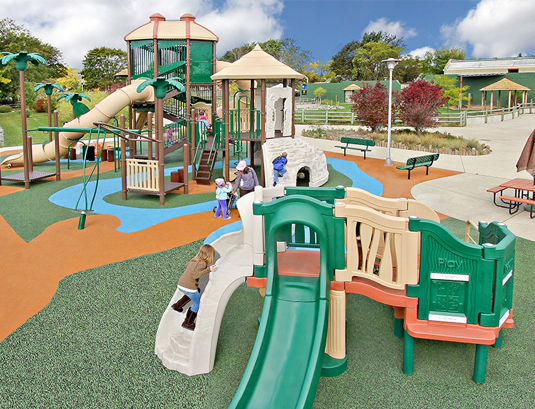The image depicts a vibrant outdoor children's playground set against a backdrop of grass and trees, with a green building partially visible in the background. The playground features multiple structures, built from a mix of metal and plastic materials. The play area is laid out on a cushioned surface in hues of greens, browns, and light blues, providing a safe environment for children.

The topmost section of the image reveals some small red trees to the right and a paved pathway that meanders in front of the green building and loops around the playground. 

Prominently in the background of the playground, there is a large playset with a long, enclosed tubular slide beginning from the second floor. This structure, composed of metal and hard plastic, is equipped with climbing areas and topped with small white roofs. Adjacent to it is a shorter but similar structure, both contributing to a two-story play area experience. 

In the mid-ground, you can see a woman kneeling with a small child to her left. They are positioned near a small white wall that seemingly leads to an entrance to one of the play structures.

The foreground is dominated by another playset, extending from just left of the middle to almost the right edge of the image. This playset features a central green slide that leads out of the frame at the bottom, with accompanying peach and green elements, including a tan piece and small stairs on the other side. To the left of this green slide is a smaller white slide, where a young child is lying face down, ready to slide down.

Further to the right, we see a couple of green benches with a light pole between them and a pink table that extends out of the image. The entire scene is brightened by a clear blue sky with scattered clouds.